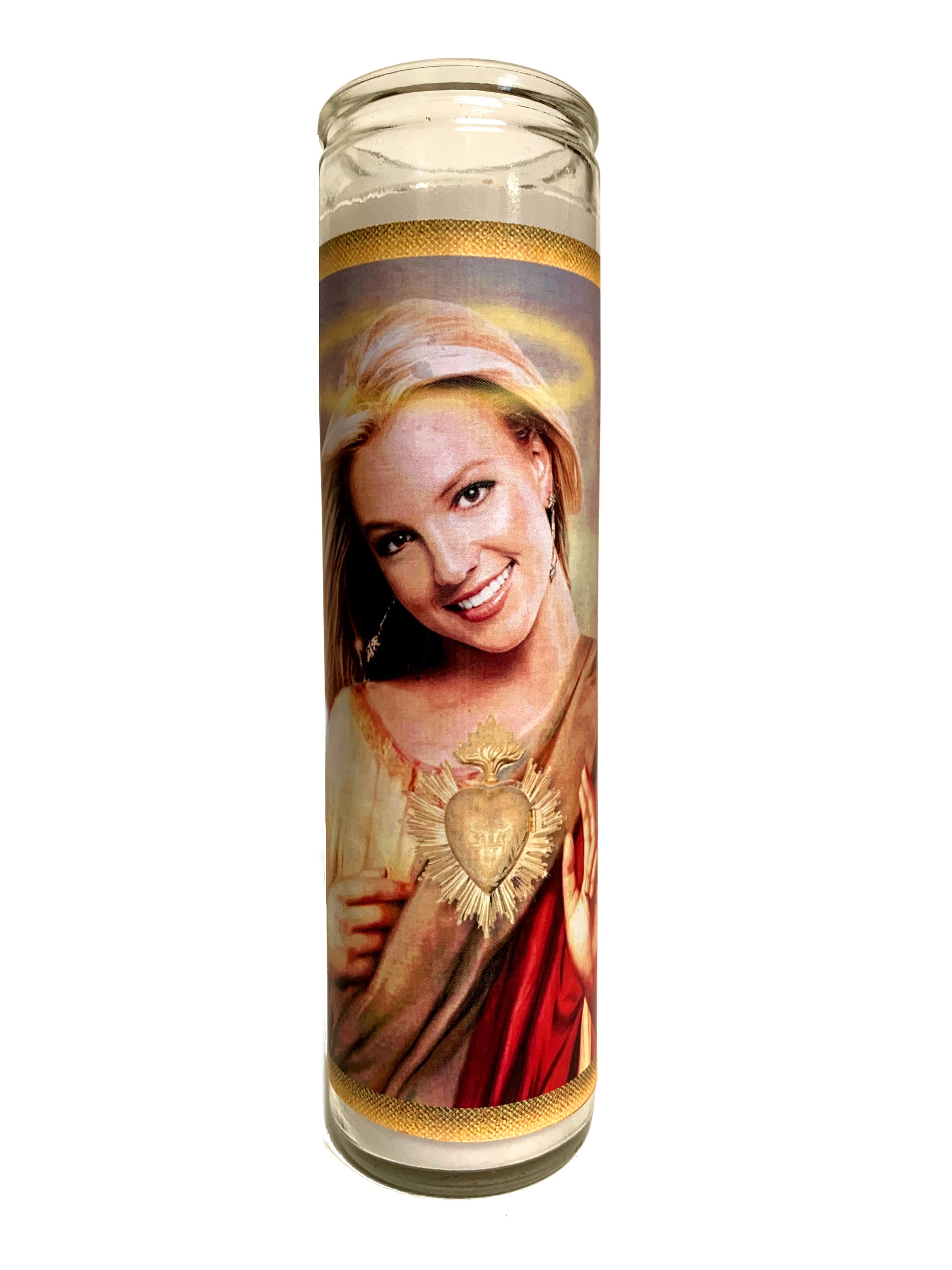The image depicts a tall glass candle, typically used for religious ceremonies, featuring a stylized picture of pop singer Britney Spears. Britney is depicted with her blonde hair pulled back, smiling brightly. She is adorned in a white and gold attire with a maroon robe draped over her shoulders, complemented by a red sash and a gold heart, surrounded by a design, pinned to her chest. Her hands are positioned near her chest; the left one is raised while the right is cupped close to her right side. She has a halo around her head, and the candle’s glass container is trimmed with gold horizontally across the top and bottom, set against a purple background with gold details.